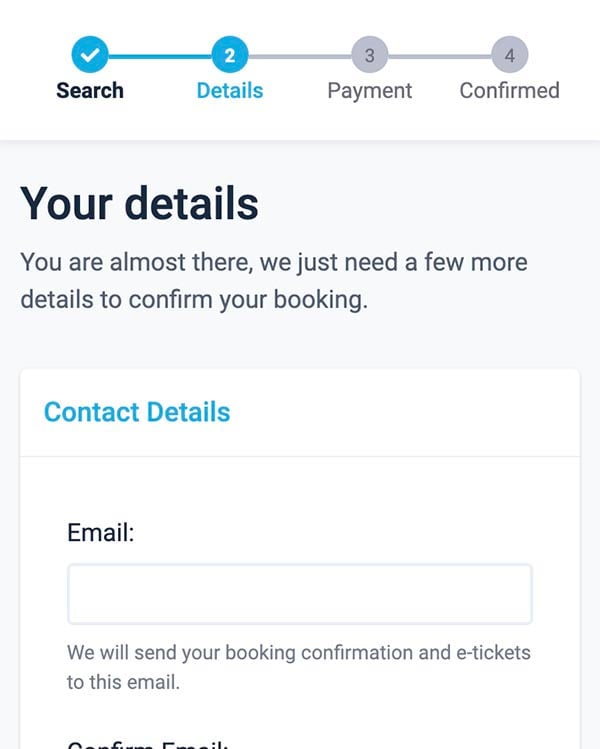"An enlarged section of a booking confirmation process is displayed. The interface features a clean and simple design with colors including white, beige, black, light blue, and gray for most of the text. The second step of a four-step process is highlighted, indicating that the user has completed their search and must now enter their contact details. A blank input box awaits the user's email address, which is crucial for sending the booking confirmation and e-tickets. The text, 'Your details,' signifies that the user is almost done and just needs to input a few more pieces of information to proceed to the payment phase, after which the booking will be confirmed. Prominently, 'Contact details' is highlighted in blue, directing the user's attention to this required field."